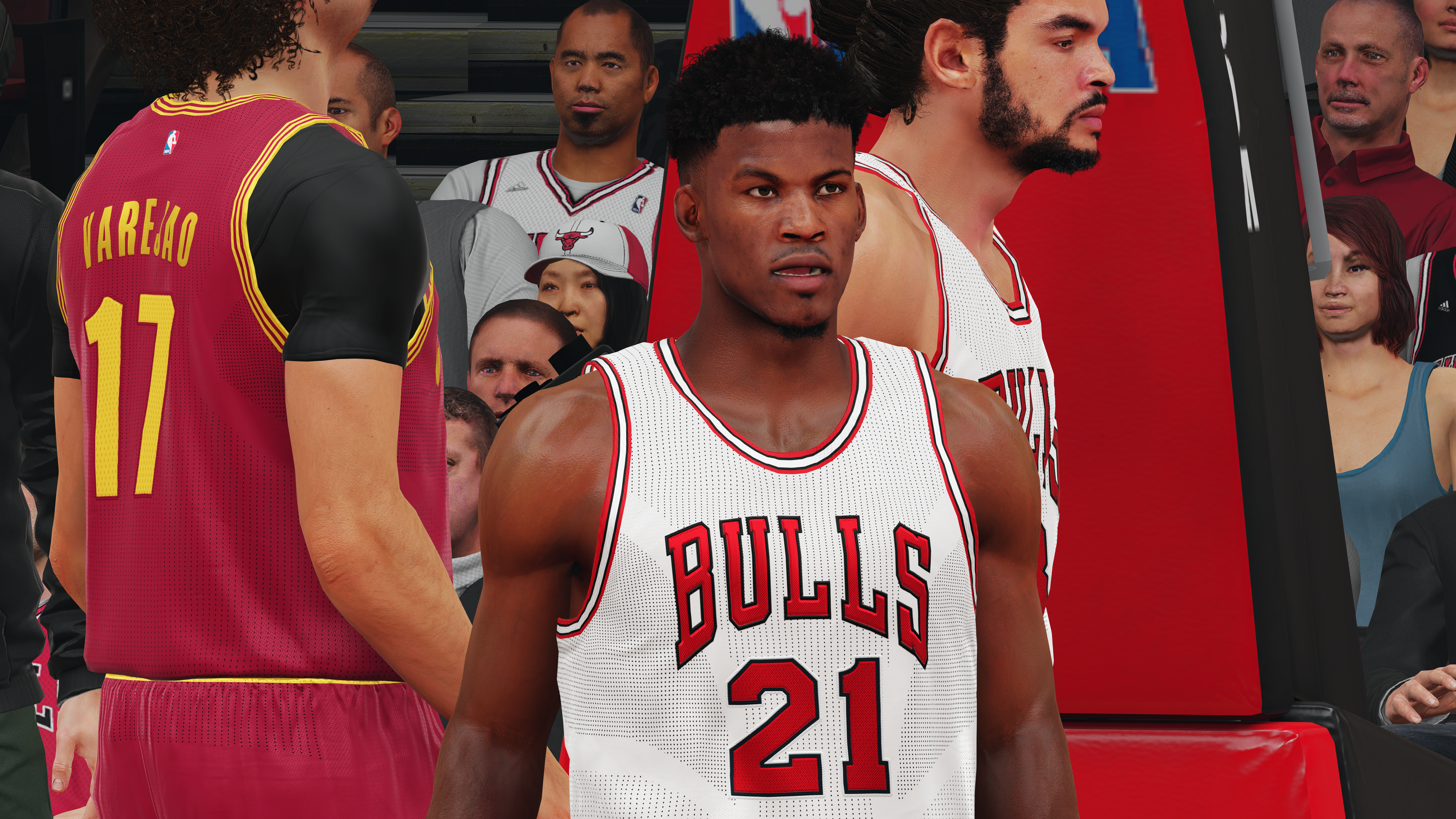This detailed caption combines and emphasizes shared details from the multiple descriptions:

---

In this nearly photorealistic video game screenshot, the central focus is a young African-American basketball player wearing a Chicago Bulls jersey with the number 21. He stands at the forefront with his mouth open, seemingly in the middle of an intense game moment. His hair is short and slightly spiky, framed by a fade on the sides, and he has minimal facial hair. Behind him, you can see another Bulls player to his right, as well as an opponent clad in a maroon, black, and yellow outfit. The opponent's jersey appears painted tightly onto his form, further signifying the image's digital origins.

The background revealing audience members seated closely to the court, especially a woman positioned behind a safety barrier under the hoop, also hints at the game's simulation nature, as the seating arrangement and expressions look unrealistic for a live event. The game's attention to detail extends to the scoreboard text displaying “Yariko 17” and “Bulls 21.” The overall color palette of the scene includes black, white, brown, red, maroon, yellow, and blue. The realism and intricate details of facial expressions and court elements confirm this image as a capture from a sophisticated basketball video game.